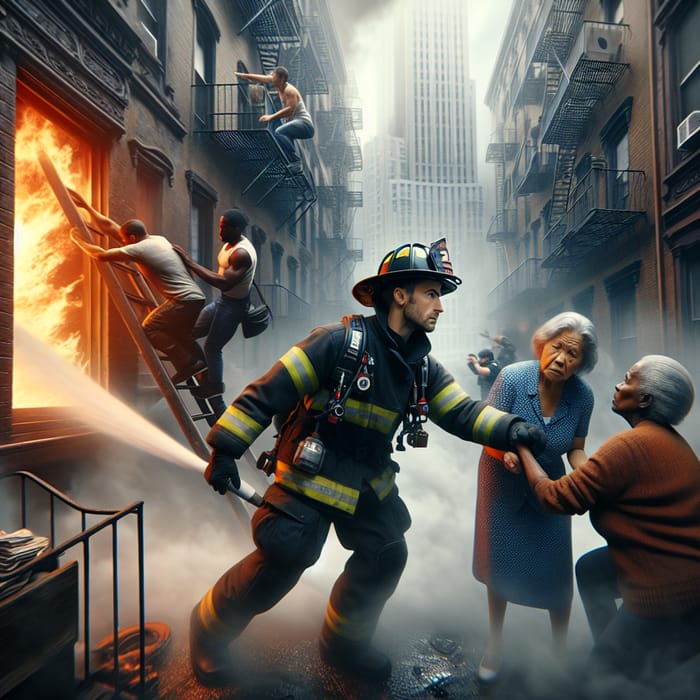In this digital illustration set in what appears to be New York City, a dramatic scene unfolds amidst a chaotic fire. Central to the image is a firefighter, distinguished by his black helmet emblazoned with a shield bearing the number 2 and yellow and white checkered squares on top. Clad in a gray fire suit with fluorescent yellow and silver stripes, he reaches out to rescue a distressed elderly black woman who kneels before him, looking up for help. Beside this woman, an elderly Asian woman also seeks his aid. Strangely, a fire hose seemingly emerges from the firefighter's leg, spraying water into a window of the apartment building engulfed in flames to the left. The street is lined with apartment complexes, and a distant skyscraper can be seen through the smoke-filled backdrop. Adding to the chaos, a civilian man descends a ladder positioned precariously against the burning structure, assisted by another black man. This image, replete with surreal and unsettling elements, captures a moment of crisis and desperate resilience in a cityscape under fire.